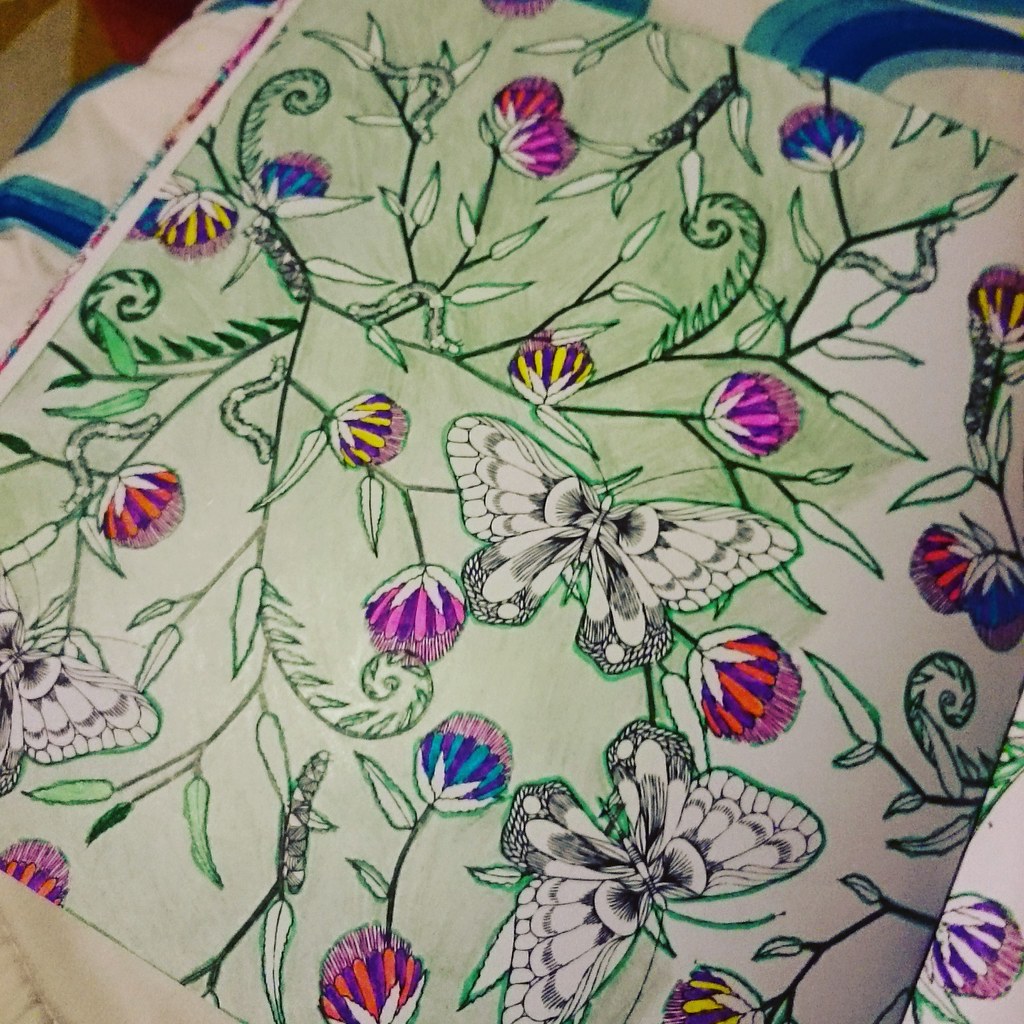A close-up of a decorative throw pillow showcases a detailed, partially colored floral design. The pillow's fabric features a predominantly green and white pattern with a mix of unopened flowers and white butterflies, creating a whimsical, yet unfinished look. The edges are adorned with a teal green and blue striped pattern, accentuated by visible seams where the fabric has been meticulously sewn together. The design appears to invite further personalization, possibly with fabric markers, as the coloring progresses from left to right without touching the butterflies. This unique, artistic pillow combines stylish aesthetics with a hands-on, creative opportunity.